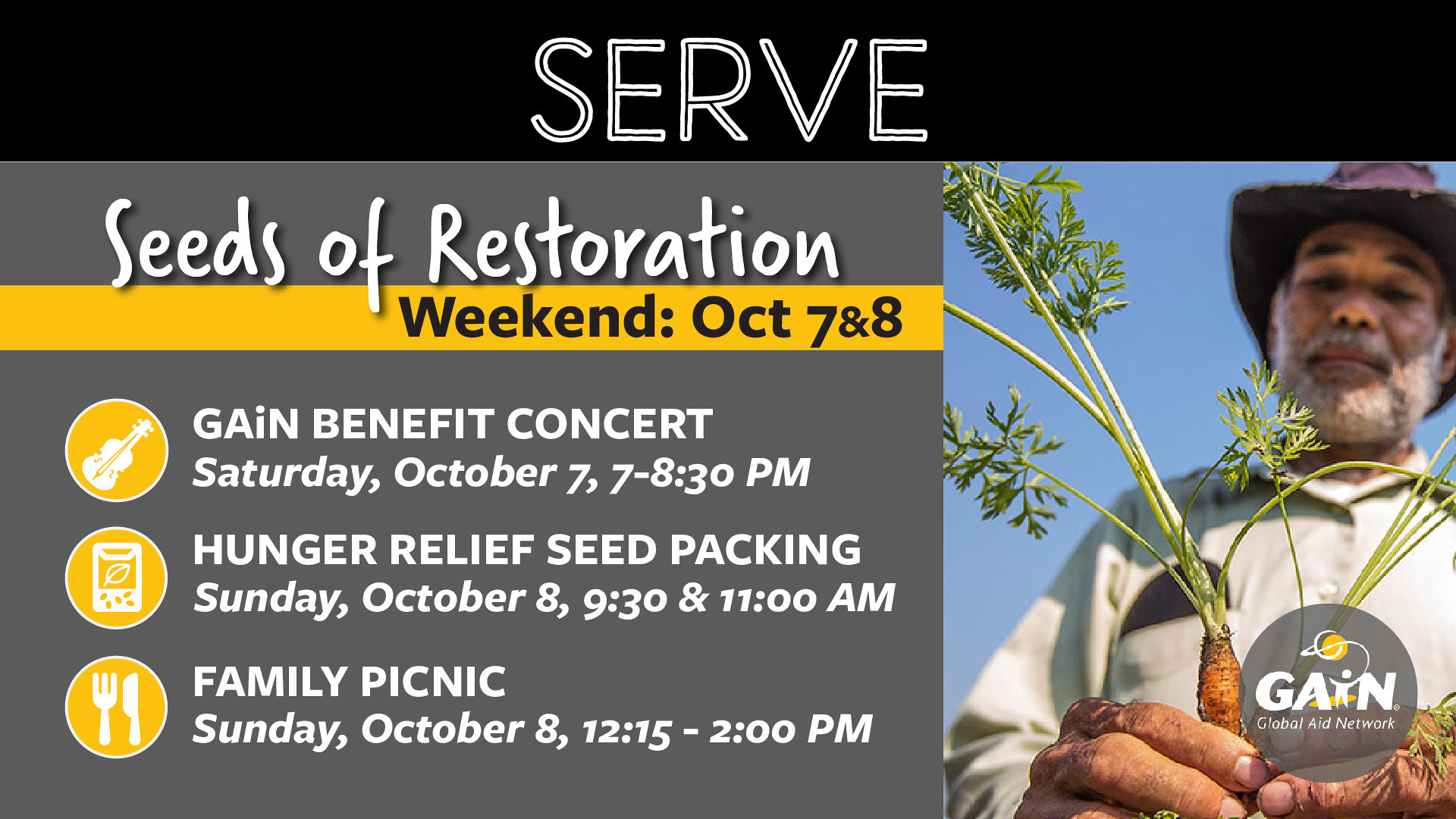This horizontally aligned rectangular image serves as an advertisement for upcoming events. Dominating the top portion is a black banner with the word "SERVE" in bold, white capital letters. Below this banner, on the left side, there is a solid dark gray rectangular section. At the top of this section, the white text reads "SEEDS OF RESTORATION." Directly beneath it, a yellow rectangle bears the text "WEEKEND OCTOBER 7 AND 8" in black. Following this are three rows of event information: a circular guitar icon accompanies "GAIN BENEFIT CONCERT, SATURDAY, OCTOBER 7, 7 to 8:30 PM" in white text; an icon for Hunger Relief Seed Packing alongside "HUNGER RELIEF SEED PACKING, SUNDAY, OCTOBER 8, 9:30 AND 11 AM"; and a knife and fork icon next to "FAMILY PICNIC, SUNDAY, OCTOBER 8, 12:15 to 2 PM."

In the lower right section of the image, there's an upward-view photograph of a man with a gray beard and mustache, wearing a purple hat and a white button-up shirt. He is intently looking down at a carrot in his hands, with bits of orange and green stems visible. Near his hands, a circular gray logo reads "GAIN," with the "i" stylized as a small person, indicating the Global Aid Network. The overall color palette of the image includes black, white, gray, yellow, green, orange, tan, brown, and purple, creating a visually cohesive and informative advertisement.